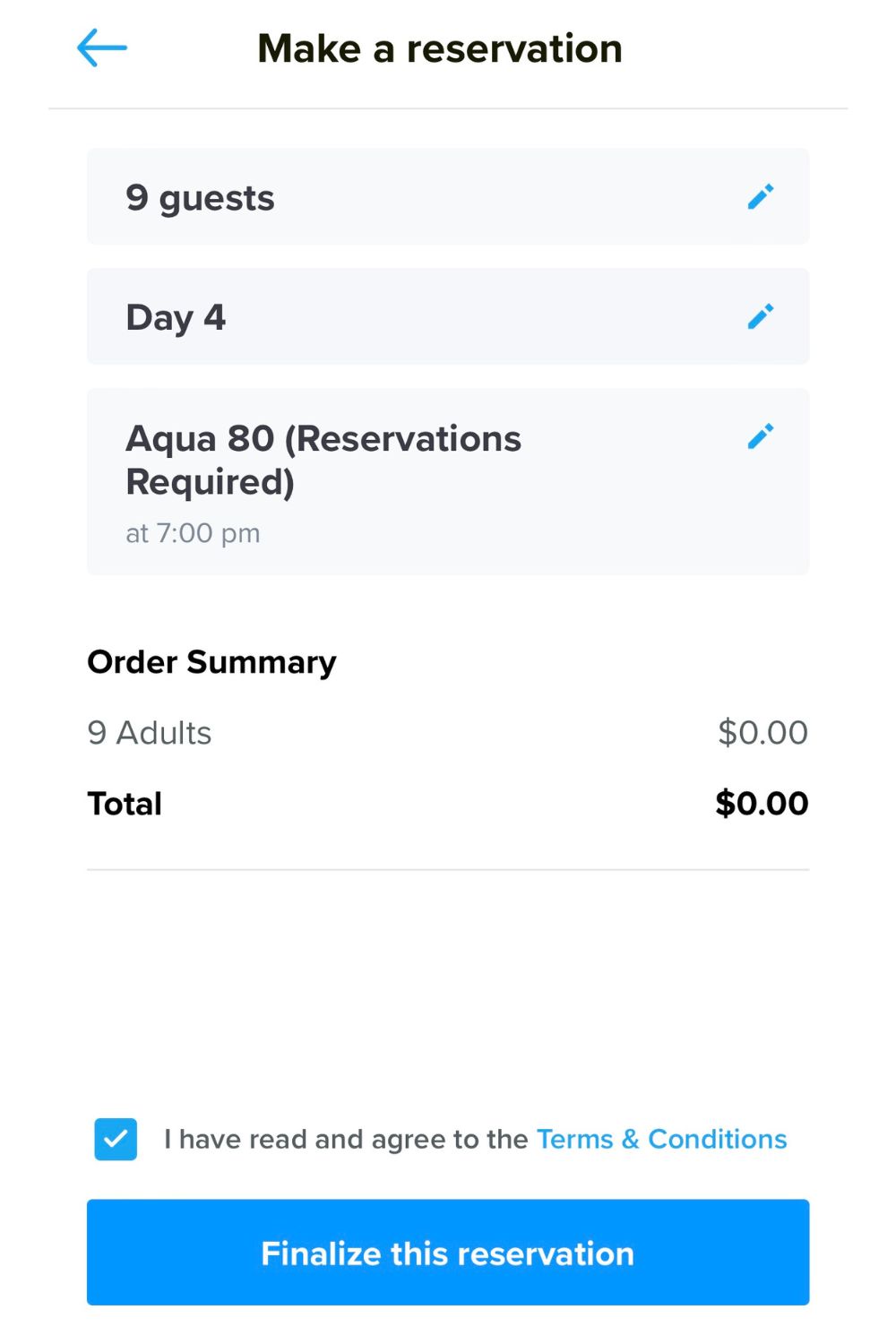The image displays a screenshot on a solid white background. At the top, bold black text reads, "Make a Reservation." To the left of this text, there's a blue arrow pointing to the left. Directly below, there is another line of bold black text stating, "Nine Guests," positioned inside a very light gray box with a blue pencil icon to the right.

Further down, the words "Day Four" appear in bold text, accompanied again by a blue pencil icon in a gray box. Just below, another gray box features the text "Aqua 80, Reservations Required at 7 p.m." with a blue pencil icon to the right.

The section beneath this contains the "Order Summary" in black text, listing "Nine Adults, $0" below it. Under this, bold text indicates the "Total: $0." 

A checked blue box follows, stating, "I have read and agreed to the terms and conditions." Finally, at the bottom, a blue box reads, "Finalize This Reservation."